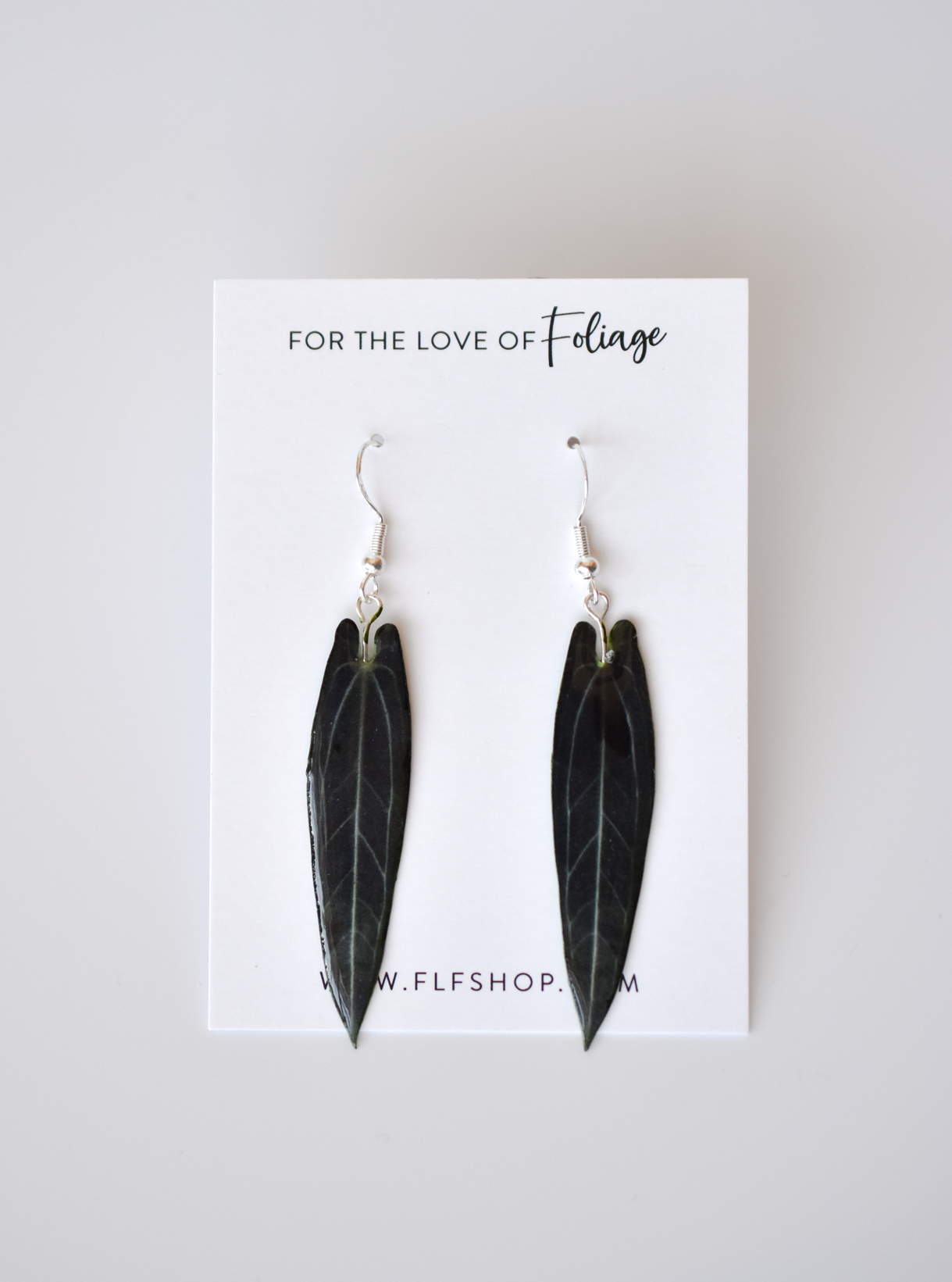The photograph showcases a pair of unique earrings displayed on a white card with the phrase "For the Love of Foliage" at the top, where "foliage" is styled in a different font. These earrings are designed to resemble elongated, pointed leaves, complete with detailed vein tracings that give them a somewhat glossy appearance. They are attached to silver hooks for pierced ears and measure approximately 1.5 to 2 inches long. At the bottom of the card, partially obscured by the earrings, is a website, likely www.flfshop.com, where one can presumably purchase the earrings or find additional matching items. This close-up color image is set against a gray square background, emphasizing the intricate details of the earrings.